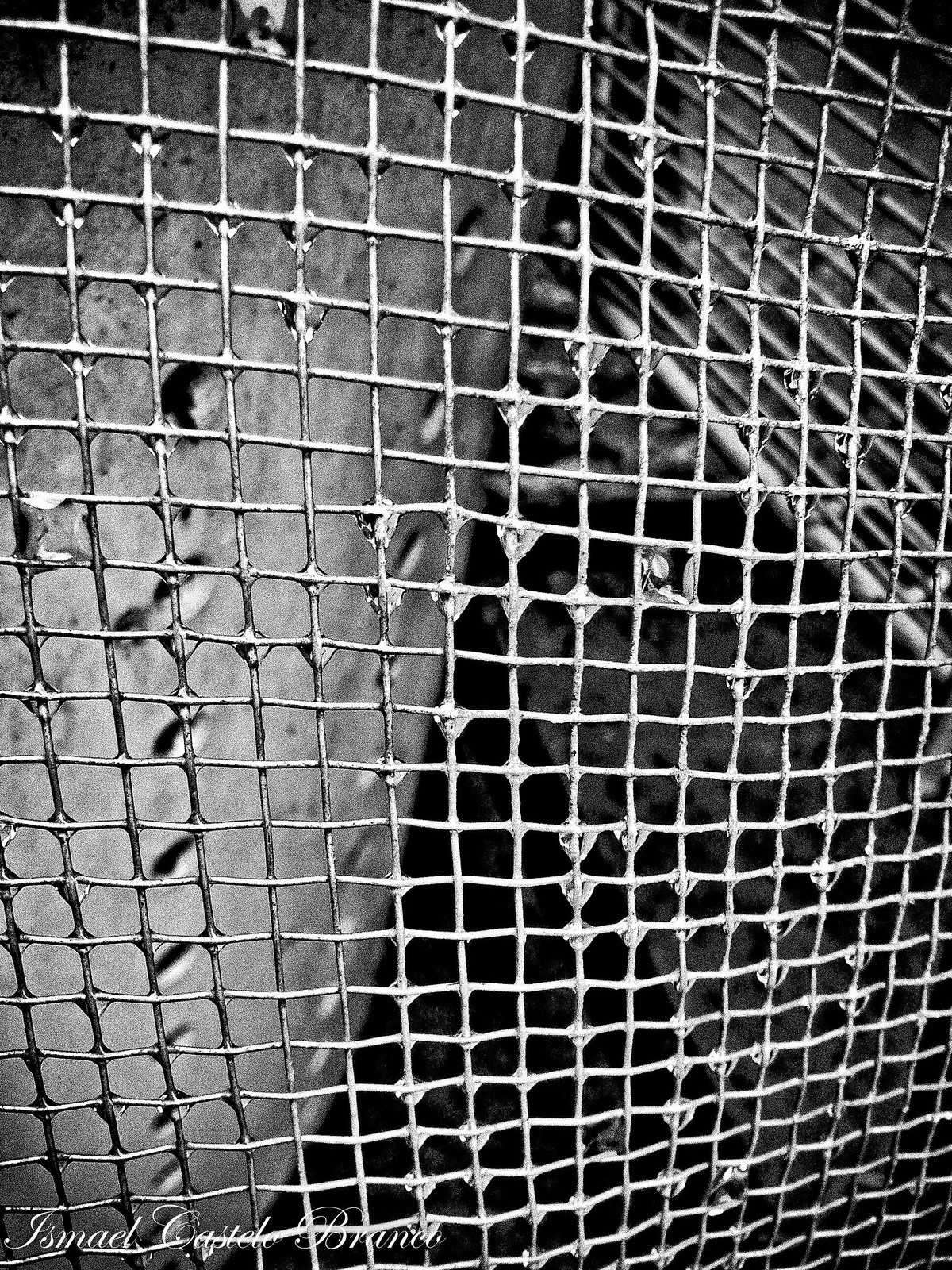This is a stark black-and-white artistic photograph taken through a metal wire fence, resembling garden or chicken wire, with interwoven silver metal wires forming small squares, approximately half an inch to a quarter inch in size. The fence is adorned with various droplets of water, hanging and dripping slightly, suggestive of recent rain. The high-contrast image captures intensely black and white elements, creating a dramatic visual effect. In the background, darker shades suggest an indistinct, murky interior. To the upper right and lower left, there appears to be another layer of fencing or a grate, adding to the complexity of the scene. The bottom of the photograph displays a watermark that reads "pommel," followed by indistinct letters "G" suggesting a signature or an artist's mark. The background is predominantly dark, making it difficult to discern the exact location, though it could imply an outdoor or industrial setting.